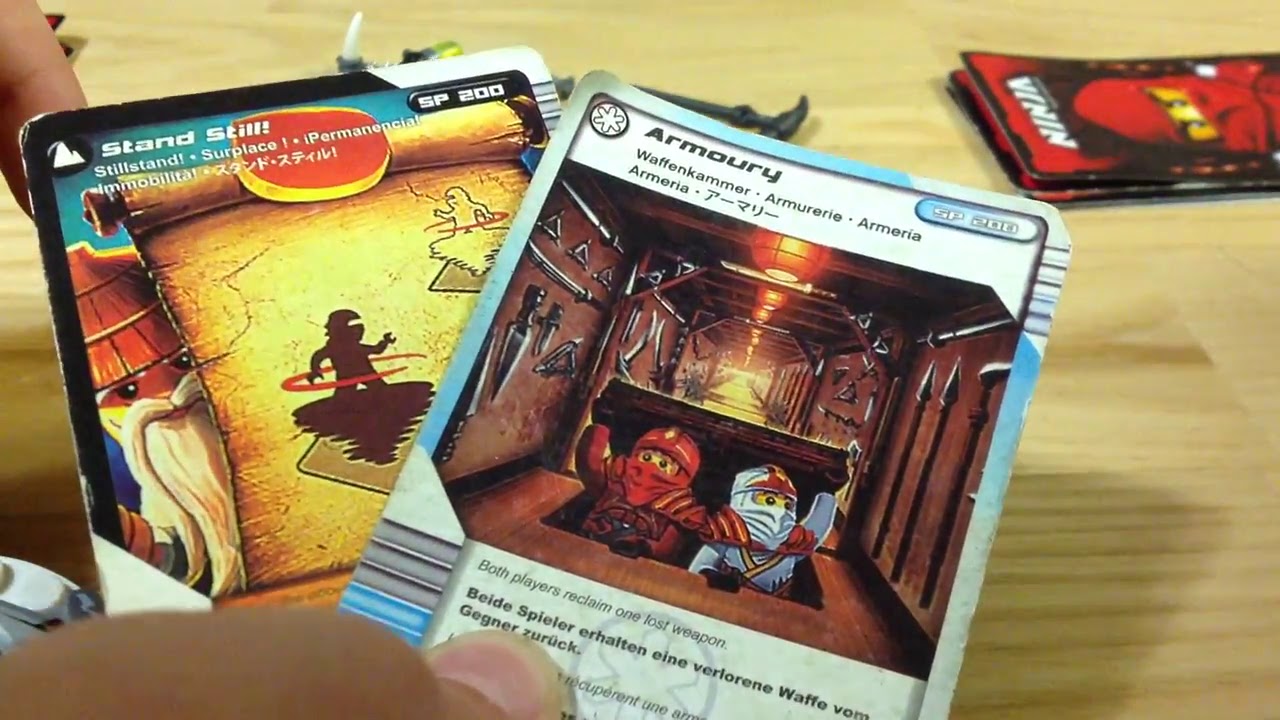The photograph captures a close-up view of a set of playing cards held in the hands of the observer, looking down onto a light wood table. In the lower left corner, a brown thumb with a visible fingernail is seen, while the upper right corner reveals the underside of a single brown index finger. In the center, two playing cards are held in a V shape, revealing details of each card. The top card is white with black text reading "Armory, Waffenkammer, Armoria," and displays two Lego-like figurines, one in red and one in white, emerging from a trapdoor into a room filled with armaments. The card beneath it, titled "Stand Still," features two ninja-like characters seemingly frozen in motion atop a tornado, with additional text in various languages such as "Surplace" and "Permanencia." The bottom card also includes a small figure in a straw hat with a flowing mustache and beard, peeking from behind a scroll. To the upper right corner of the image, two more cards lay horizontally, one labeled "Ninja" with an image of a red ninja Lego figurine.